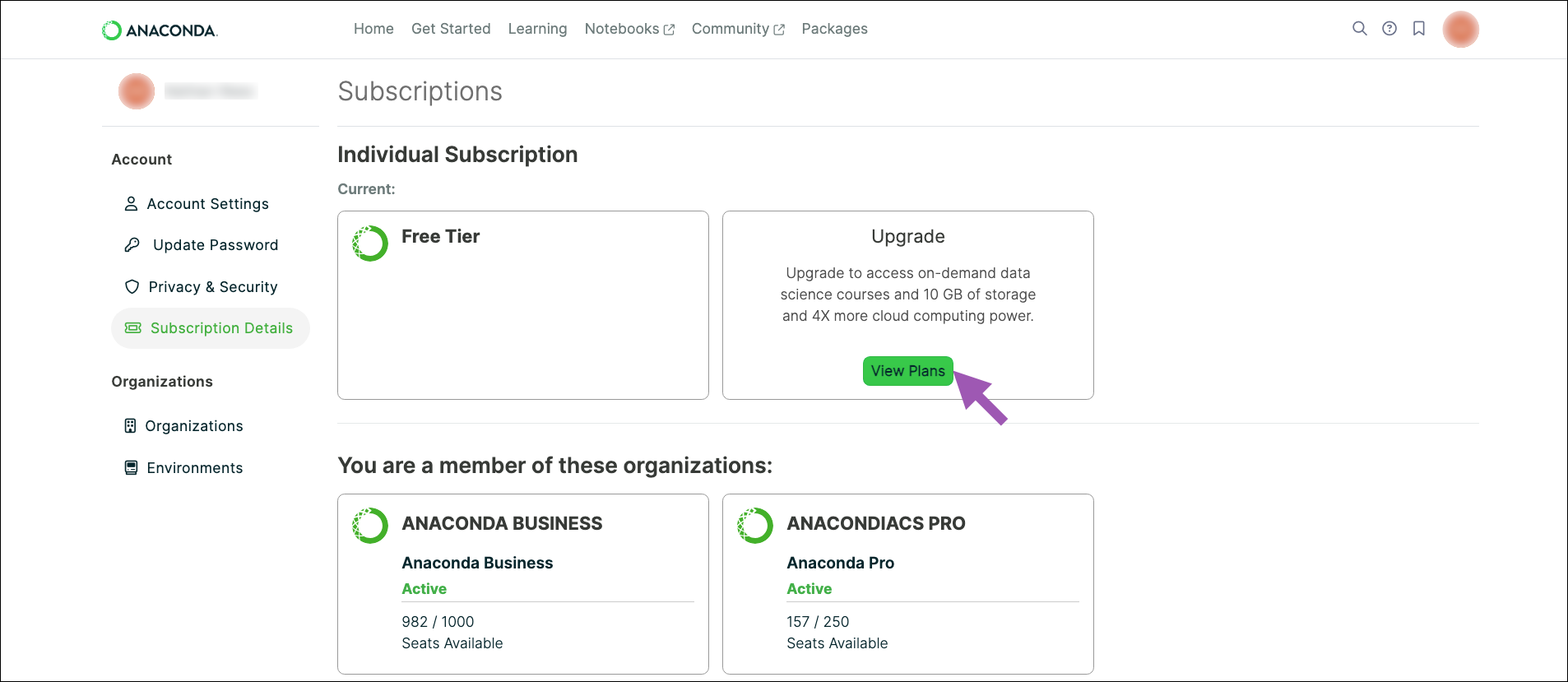This is a detailed screenshot from the Anaconda website, which highlights various subscription options and membership details. The screenshot displays Anaconda's individual subscription plans, including a free tier and a paid upgrade option. The upgraded plan offers around 10 gigabytes of storage and four times more cloud computing power, albeit at a higher cost. To emphasize this paid upgrade, a pink arrow has been digitally added to the image, likely to prompt the user to consider purchasing the upgrade.

Additionally, the screenshot reveals that the user is a member of two separate organizations: "Anaconda for Business" and "Anaconda Pros." The "Anaconda Pros" account currently has 157 out of 250 seats available, while "Anaconda for Business" has 982 out of 1000 seats available, indicating ample space for users. On the left-hand side of the screen, there are further account settings options for navigation.